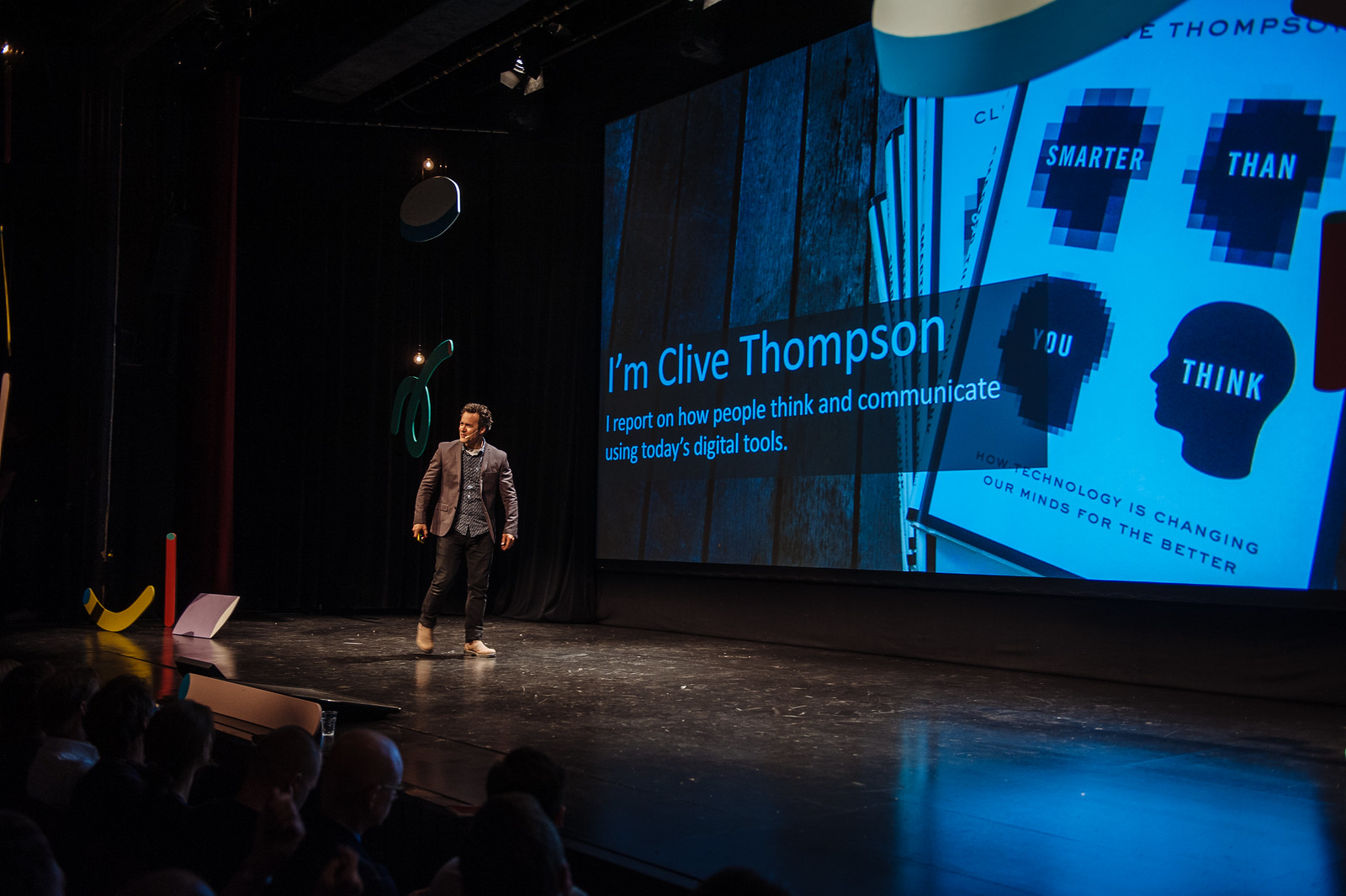In this detailed color image, we see Clive Thompson walking confidently on a large stage, illuminated by a spotlight, giving the impression of a TED Talk or book promotion event. He is casually dressed in a light tan jacket over a dark shirt, paired with black pants and beige shoes. Clive has brown hair with a high forehead line and is smiling at the audience, adding a welcoming atmosphere to the scene.

Behind him, a large screen prominently displays a light blue text introducing him: "I'm Clive Thompson. I report on how people think and communicate using today's digital tools." To the right of this text, the screen features a book cover with pixelated images of a human head progressively getting clearer, visually representing cognitive enhancement. The words "Smarter Than You Think: How Technology is Changing Our Minds for the Better" are clearly visible, indicating the theme and title of his book. The background of the stage includes some dim lighting and scenery elements, enhancing the professional setting and focus on Clive's engaging presentation.